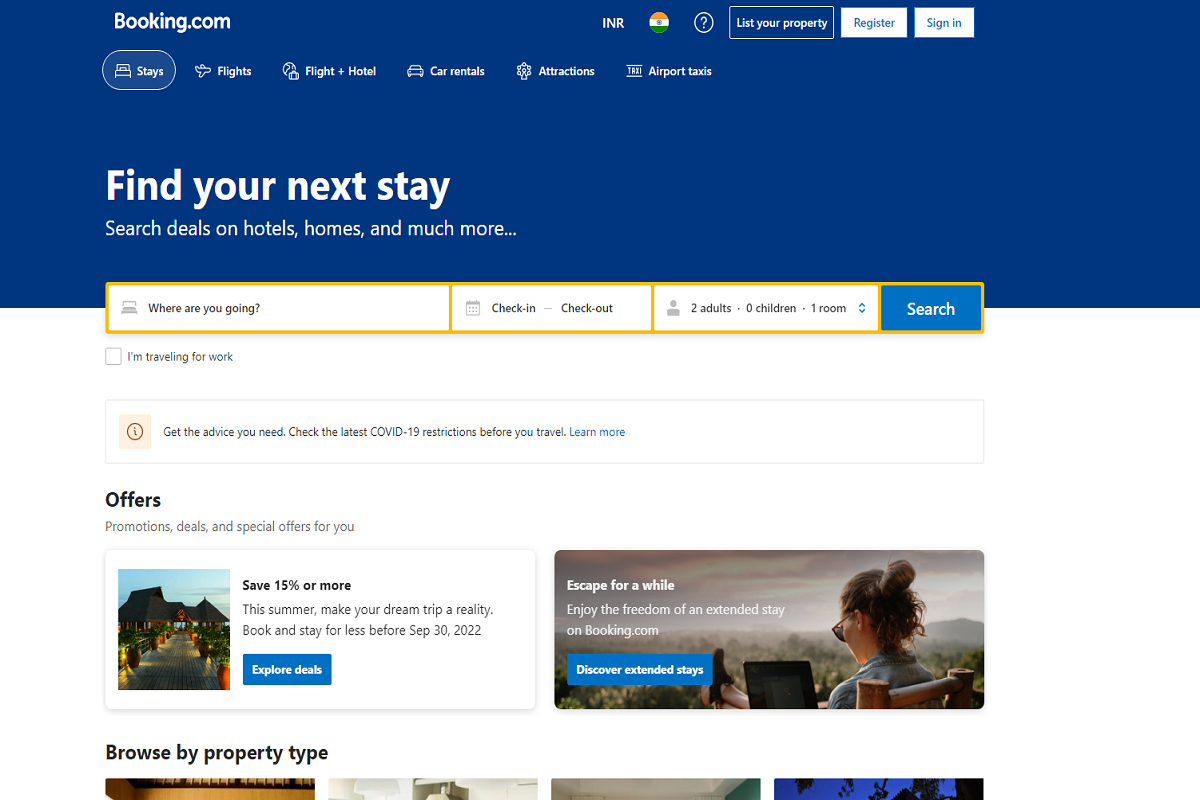Screenshot of the Booking.com Homepage

The image portrays the upper segment of the Booking.com website interface. Dominating the top portion is a slightly darker-than-royal-blue rectangular banner. Within this banner, click-able options are neatly displayed, including "Stays," "Flights," "Flight + Hotel," "Car Rentals," "Attractions," and "Airport Taxis." An INR currency section is also visible, denoted by a circle bearing the colors orange, white, and green. To the right, options for "List your property," "Register," and "Sign in" are available.

Prominently positioned below the banner is a welcoming message in bold text: "Find your next stay. Search deals on hotels, homes, and much more." Beneath this message lies the search functionality, featuring fields such as "Where are you going?" and options to input check-in and check-out dates. Displayed details include "2 adults, 0 children, 1 room," all adjustable with ease. The search area is bordered in yellow, with a distinct blue search button for initiating queries. 

Additionally, a check-box marked "I'm traveling for work" is visible, providing users with tailored options. Further down the page, a section displays various offers and images related to travel accommodations and deals.